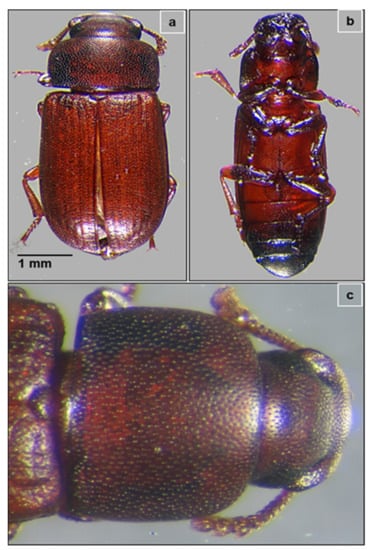This image, arranged in a portrait orientation, features three distinct close-up photographs of a brown beetle, each labeled for clarity. The upper half of the image is divided into two smaller panels. The top left panel, labeled 'A,' displays the dorsal view of the beetle, showcasing its brown coloration, two small antennae, multiple legs, and partially opened wings laid against its back. The top right panel, labeled 'B,' presents the ventral view, offering a detailed look at the beetle's legs and the dark brown to black transition near the end of its body. The larger panel at the bottom, labeled 'C,' is a close-up of the beetle's head and thoracic region, highlighting its eyes and antennae further. The background for all photographs is a uniform light gray, enhancing the beetle's features.